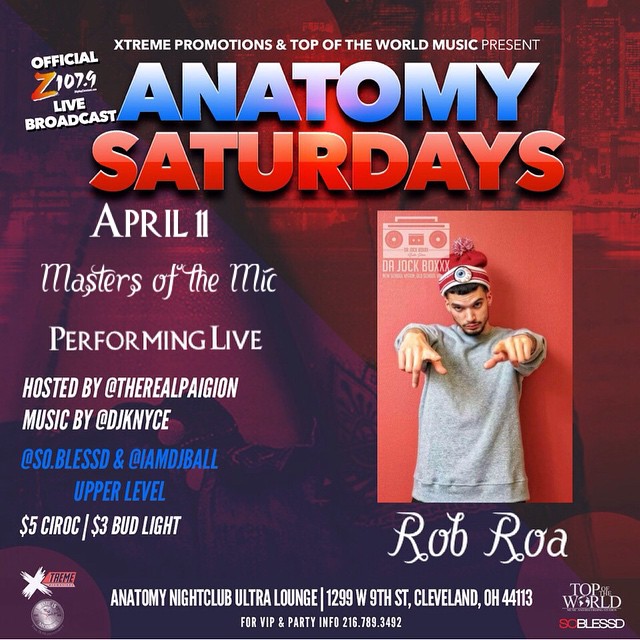An event preview poster for "Anatomy Saturdays," presented by Xtreme Promotions (spelled without the initial 'E') and Top of the World Music. The event is scheduled for April 11th. The poster features a vibrant mix of colors and text elements:

- At the top, in white text, it reads "Xtreme Promotions and Top of the World Music Present."
- Just below this, "Anatomy" is highlighted in blue text.
- Below that, "Saturdays" appears in orange text.
- On the left side, in white text, it lists the date "April 11," followed by "Masters of the Mic" in cursive.
- The event promises live performances and is hosted by @TheRealReal, with music by @DJKNYC, @So.Blessed, and @IamDJBall.
- The event takes place on the "upper level."

On the right side of the poster, an image of a man wearing a hat and a gray sweatshirt, pointing towards the camera, is featured. The man is identified below the image as "Rob Roa."

At the bottom of the poster, in detailed white text, the venue is specified: "Anatomy Nightclub Ultra Lounge, 1299 West 9th Street, Cleveland, Ohio 44113."

Pricing details on the left side note $5 for Sirach and $3 for Bud Light.